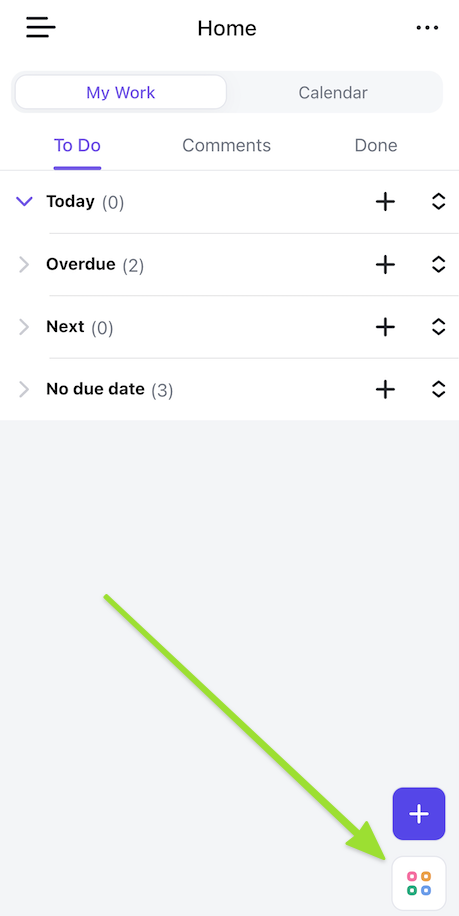The screenshot is taken from a smartphone interface with a white background. At the top center, the word "Home" is displayed in black font. On the right corner, there is a set of three horizontal dots, while the left corner features three horizontal lines, likely indicating a menu.

Below this, the screen is divided into sections. On the right side, against a very light gray background, the word "Calendar" is written in gray font. On the left side, "My Work" appears, also against a white background. Further down, "To Do" is written on the left and underlined, though there's a space between the text and the underline. Next to "To Do," there is the word "Today" in black font, followed by a downward-pointing arrow and "(0)" in parentheses.

The interface is split into three columns: "To Do" on the left, "Comments" in the center, and "Done" on the right. Opposite the "Today" section, there's a plus sign and two arrows (one pointing up, the other down).

Additionally, three items are listed under "To Do": 
- "Overdue" with "(2)" in parentheses
- "Next" with "(0)" in parentheses
- "No Due Date" with "(3)" in parentheses

Below these items, there's a very light gray square featuring a green arrow pointing diagonally down-right. Within this square is a white shape containing four circles—two blue on top and two red below them—and above this is a purple square with a white plus sign.